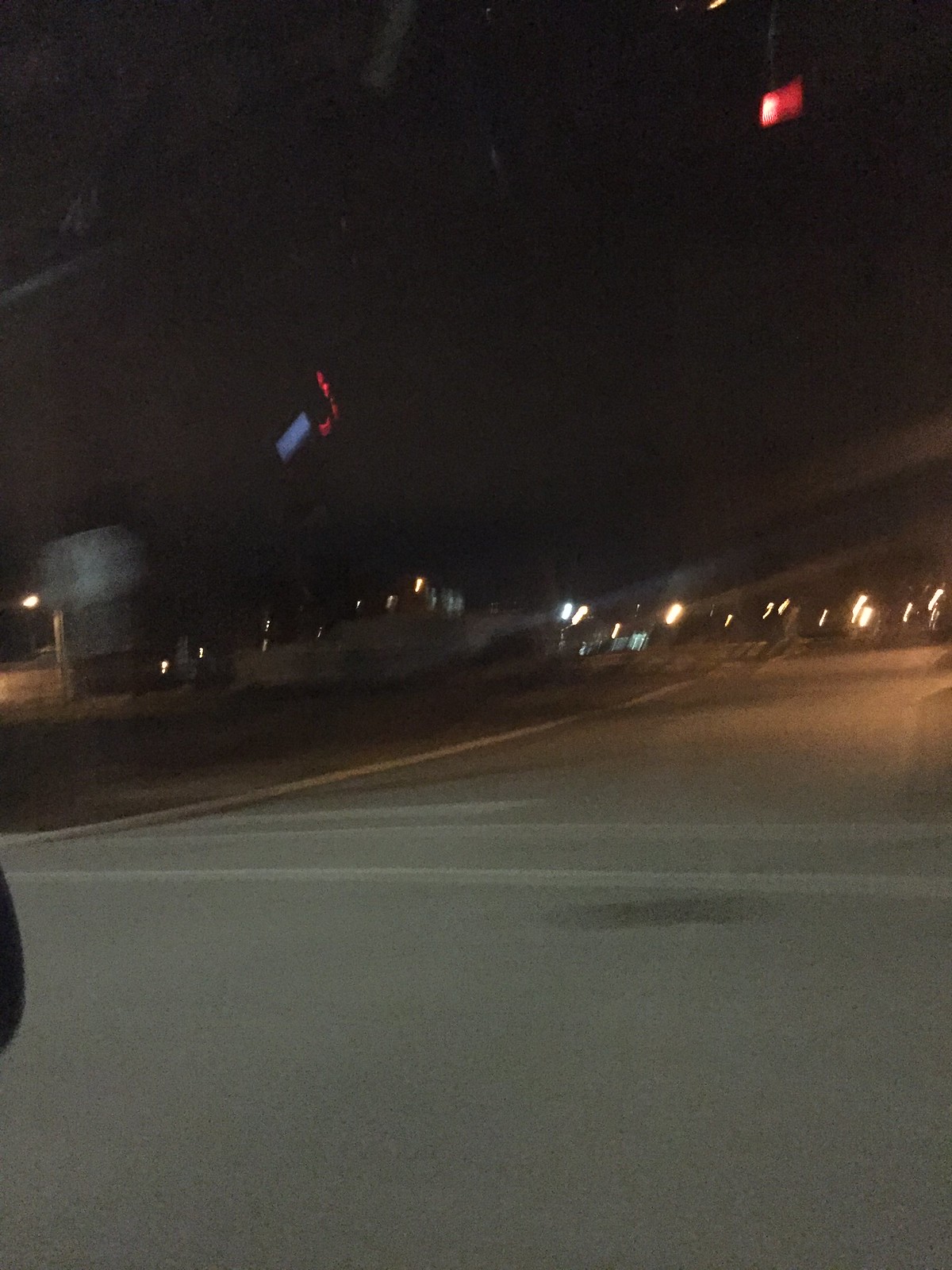A nighttime photograph taken from inside a moving car, capturing an empty road shrouded in darkness. The blurred image, likely due to the motion of the vehicle, conveys a sense of speed and solitude. Prominently reflecting off the car window are two striking red lights, adding a hint of mystery and depth to the otherwise void landscape.